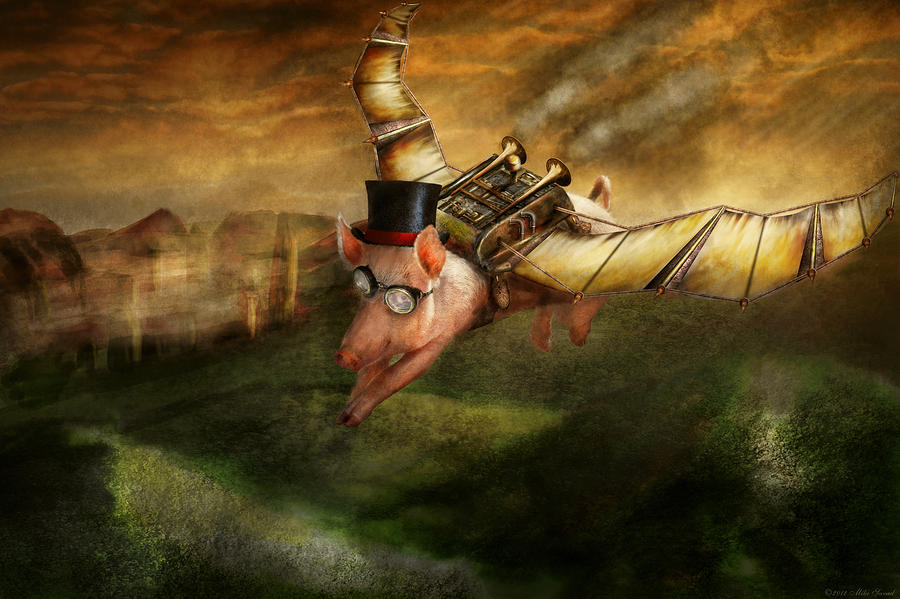This detailed illustration depicts a whimsical scene of a pig soaring through the sky, embodying the metaphor "when pigs fly." The pig, dressed in a black top hat with a red sash and sporting protective goggles, flies diagonally towards the bottom left-hand corner of the image. Large wings emerge from a backpack fixed on its back, from which brass-looking tubes resembling trumpets emit plumes of smoke. The pig's front legs are clasped together while its back legs dangle freely in the air. 

Beneath the pig, the landscape features dark green rolling hills with muted hues of green, light green, and white, suggesting a lush but subdued terrain. In the background, small houses dot the dark, brown hills and mountains. The upper half of the scene showcases a cloudy sky, painted with muted shades of orange and gray, adding to the overall dark ambiance of the artwork. The pig's head is illuminated by a bright light on its right side, which contrasts with the predominantly dark and cloudy sky, enriching the breathtaking and imaginative atmosphere of the illustration.